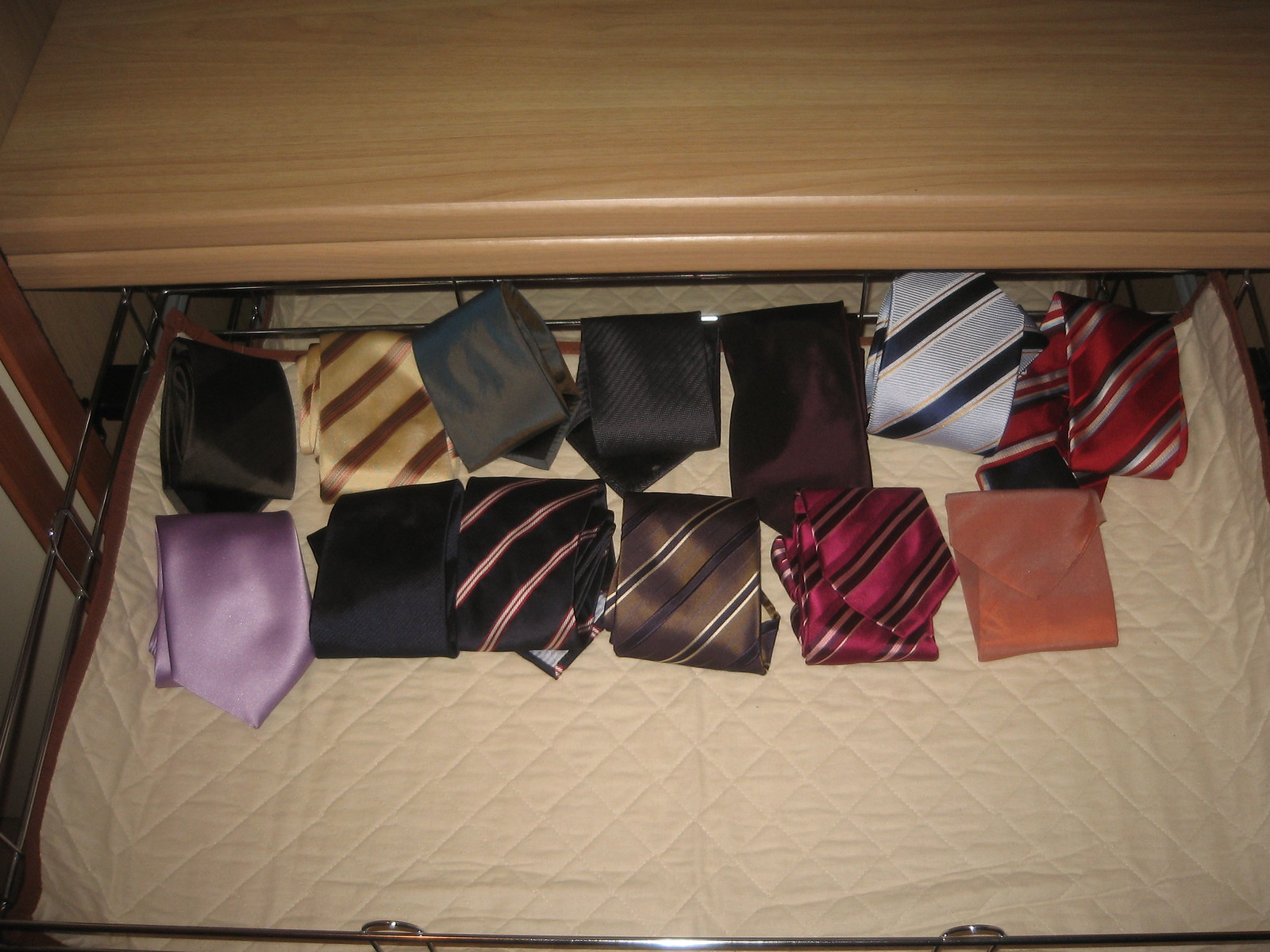The photograph features the top half of a light tan-colored piece of furniture with an opened drawer beneath it. This drawer, lined with a piece of tan quilted material, holds two meticulously organized rows of folded ties. The ties, each arranged in neat squares, come in a variety of colors and patterns.

In the front row, positioned closer to the camera, are six ties: from left to right, there's a lilac-colored tie, a black tie, a black and gold striped tie, a gold, light brown, and dark brown striped tie, a red, black, and cream-colored striped tie, and an orange tie that appears burnt in shade.

The back row contains seven ties: a brown tie, a golden-brown tie, a lighter brown tie, a darker brown tie, a rust-brown colored tie, a white and black diagonal striped tie, and on the far right, a red, black, and gold striped tie. The ties exhibit a mix of solid colors and striped patterns, underscoring the detailed and organized nature of the drawer's arrangement.